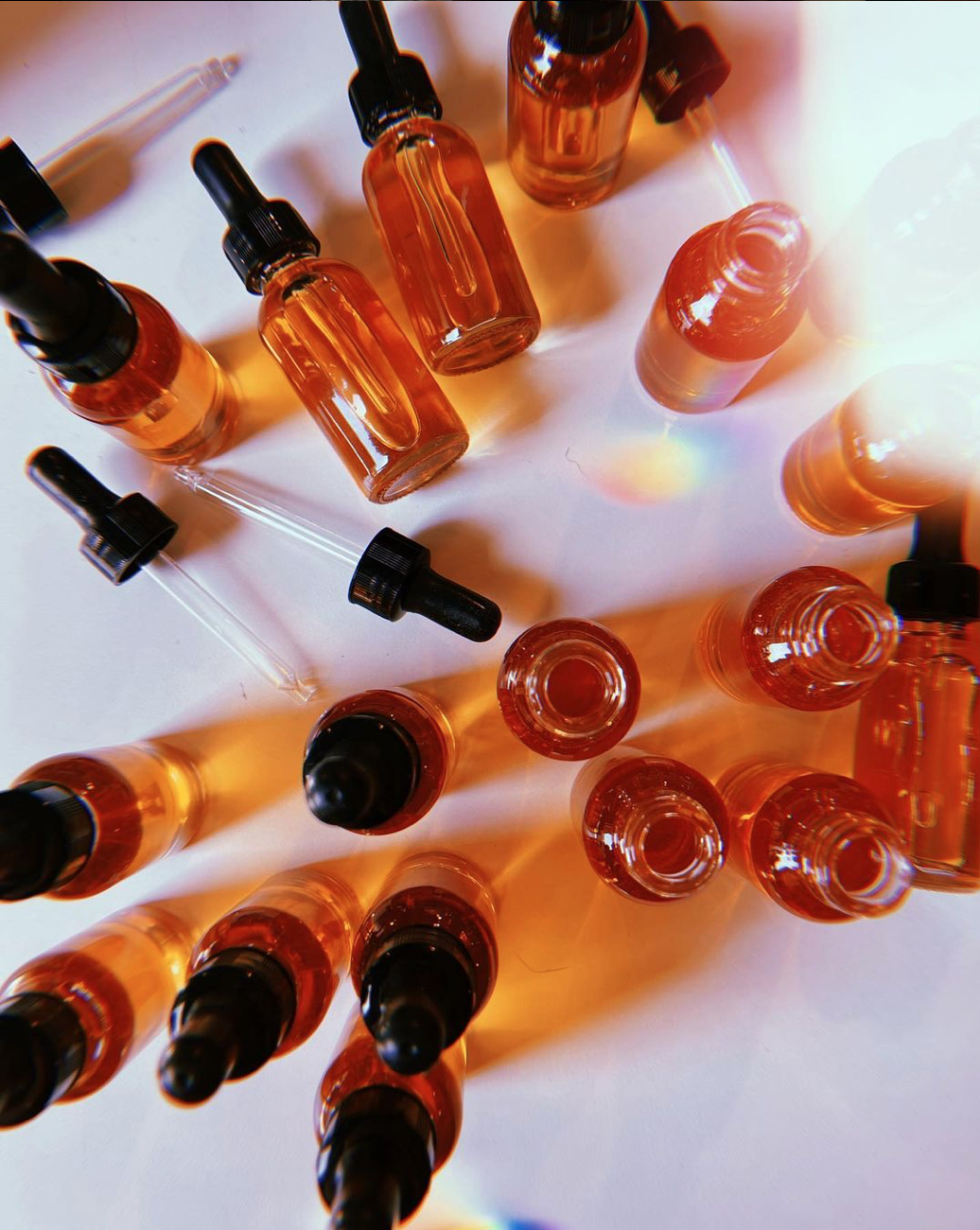In this photograph, we see a top view of small, transparent, amber-colored serum bottles placed on a plain white surface, creating the background of the image. The bottles contain a red liquid and are equipped with black twist caps that have attached clear eye droppers. Some bottles are standing upright while others are lying down, with a few caps removed and the droppers scattered around. The surface reflects an orange-yellow hue from the liquid, adding a warm tint to the scene. The upper right part of the image is slightly faded due to bright light, adding a subtle border. The diverse arrangement of the bottles and droppers, along with the reflections, create an intricate display.